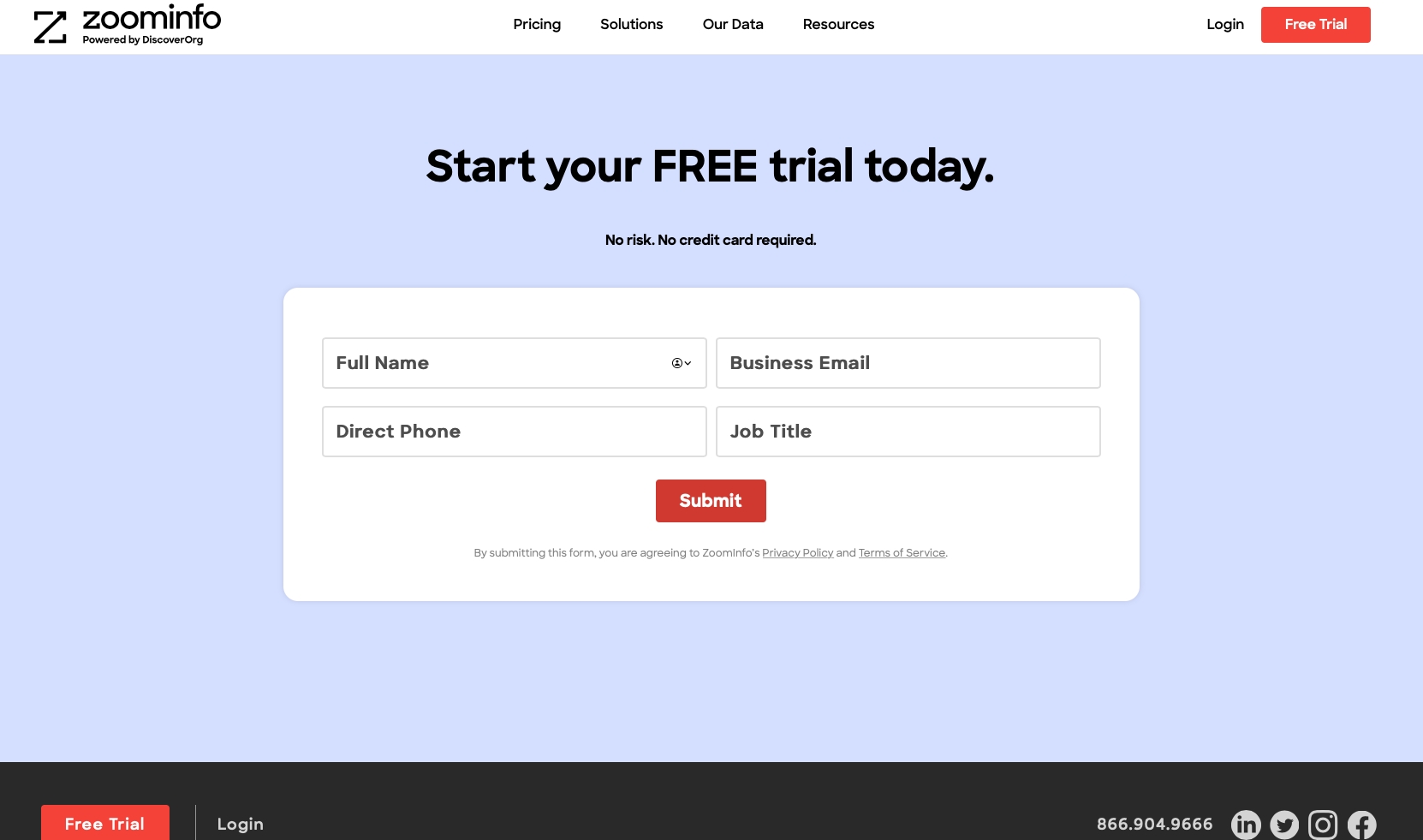Screenshot of the ZoomInfo website interface. At the top left corner, the text "ZoomInfo powered by DiscoverOrg" is displayed in black, accompanied by a distinctive "Z" logo. Centrally aligned at the top, four navigation tabs are visible, labeled from left to right: Pricing, Solutions, Our Data, and Resources. On the top right side, there are two additional tabs marked Login and Free Trial.

Dominating the central area of the image are the prominent words "Start Your Free Trial Today," followed by the assurances "No Risk, No Credit Card Required." Below this section, the page is divided into two columns of input fields. The left column includes fields labeled "Full Name" at the top and "Direct Phone Number" below it. The right column features fields for "Business Email" at the top and "Job Title" underneath.

The overall layout presents a clean and straightforward design aimed at encouraging users to initiate a free trial effortlessly.